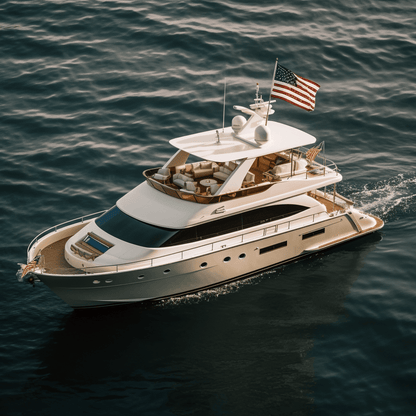This is a detailed aerial photograph, likely taken by a drone, of a luxurious multi-tier yacht cruising through dark blue, lightly rippled ocean waters, with no horizon visible, making the sea the entire background. The yacht, which appears to have at least two or three levels, features sleek gray paneling on the exterior hull and predominantly white, rounded decks. The lower level boasts large, dark-tinted windows forming the main enclosed cabin, while the upper deck, designed for entertainment, is open-air with white upholstered couches, tables, and cushions, all atop wooden flooring. An American flag flutters near the radar array and antenna on the roof. The vessel's motion creates a noticeable jet stream of churned white water at the rear, adding to the dynamic presence of the scene. The overall lighting suggests it could be taken around sunset, with soft illumination and potential sun glare, giving the scene a serene yet vibrant ambiance.